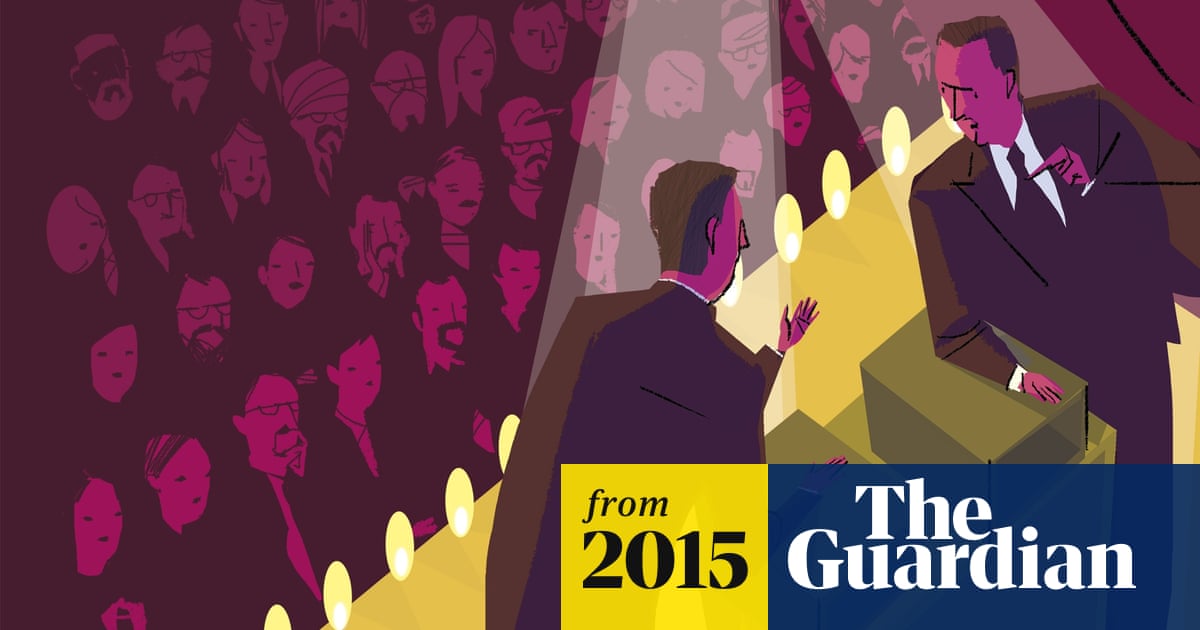The image is a stylized, cartoon-like graphic, likely from a newspaper or magazine, with branding indicating it is from The Guardian, 2015. The Guardian's logo is in white text on a blue block, next to a yellow box with the black text "from 2015." The left side of the image features an audience depicted entirely in pinkish magenta and shaded in dark purple. On the right side, a stage is illuminated with small lights lining its front edge. Two men, also colored in a pinkish magenta with dark brown hair and dressed in purplish suits, stand at podiums under spotlights that extend from the top center to the left side. They are engaged in a debate amidst a magenta-shaded crowd, all portrayed in a corporate art style.